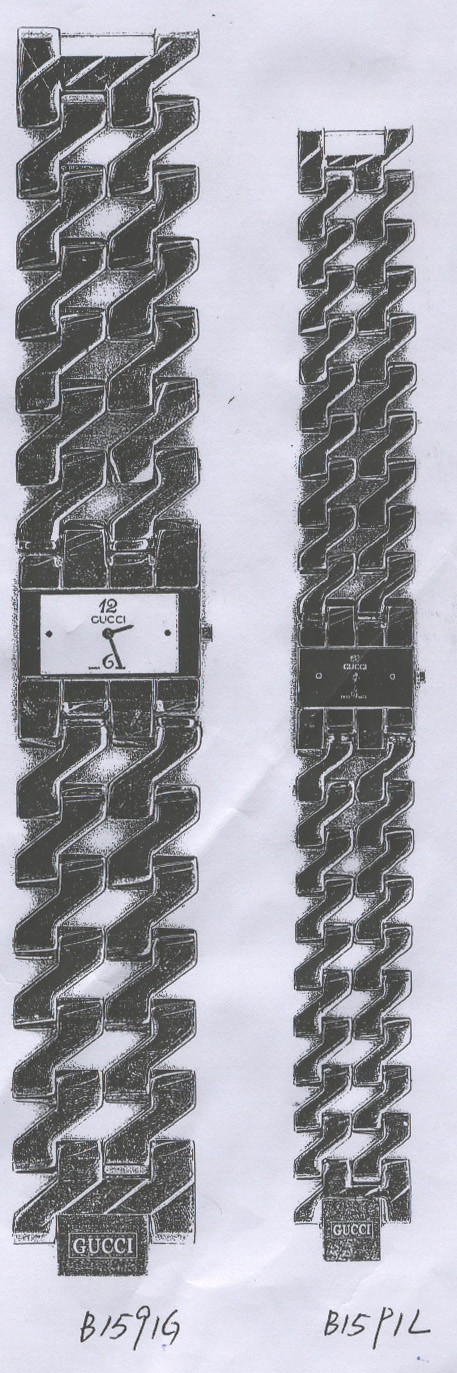The image depicts a black and white pencil drawing of two Gucci watches, organized vertically on what appears to be a patent-like diagram. The drawing features both a front and a back view of the watches. The left watch is noticeably larger than the right one. Each watch sports a rectangular clock face; the larger watch's face is white with black numbers indicating 12 and 6, while the smaller watch's face is black with golden numbers. Both watch faces exhibit two dots marking what would be 3 and 9 o'clock positions.

The bands of the watches are composed of interconnecting metal links, forming a pattern similar to black zigzags that curve and connect, creating gaps through which the skin would be visible when worn. The larger watch's links are described as being thicker and longer compared to the smaller watch's. Additionally, at the bottom of the image, there are labels: the left one reads "B15 916G," and the right one reads "B15 PIL."